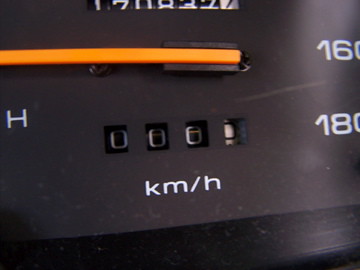This close-up photograph showcases the intricate details of a vehicle's speedometer, prominently set against a black background. The speedometer's needle is a vivid orange, immediately drawing the viewer's attention. Encircling the base, white lettering indicates the measurement in "KM/H" (kilometers per hour). Above this, a rolling number display shows a current reading of "0000." To the left of the dial, a capital "H" is positioned, with the gauge needle pointing directly above it, indicating a zero reading. Although partially obscured, the mileage counter above the needle appears to contain seven digits. On the right side of the speedometer, partially visible numerals "160" and "180" hint at higher speeds, with the zeros slightly cropped out of the frame. This detailed photograph captures the meticulous design and functionality of the speedometer, highlighting both its aesthetic appeal and instrumental precision.